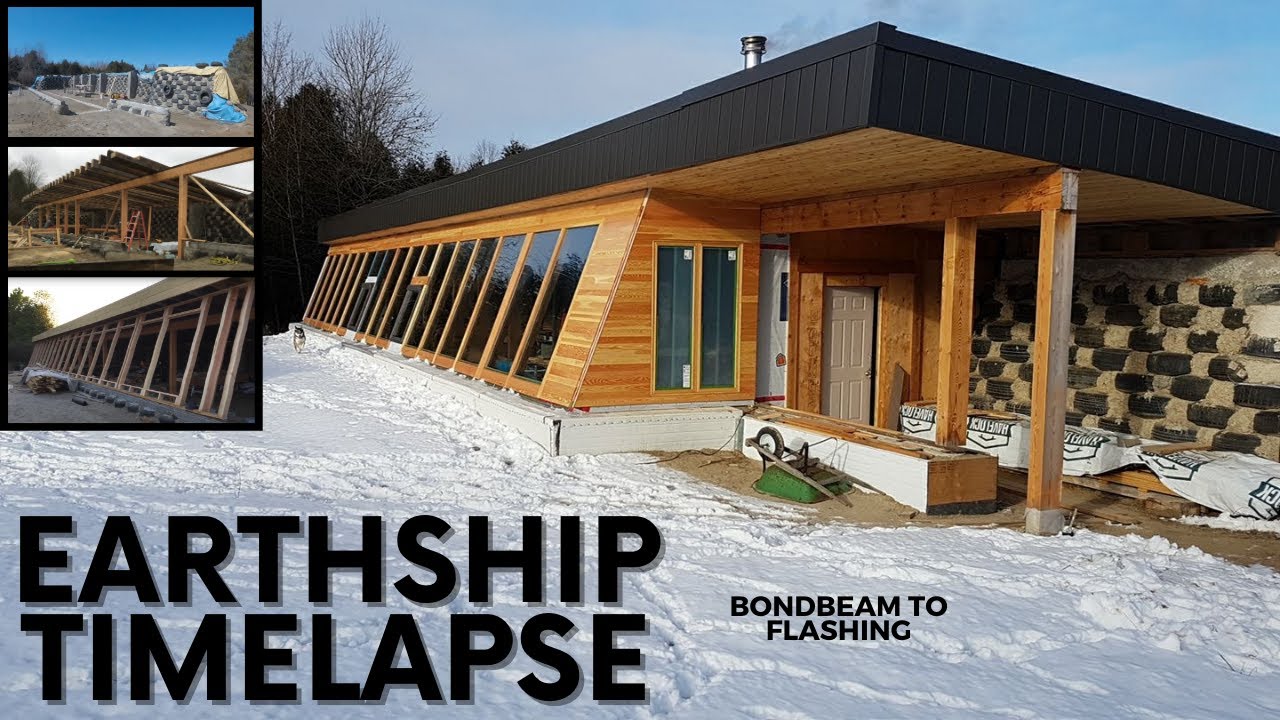This image depicts a house under construction, set against a snowy backdrop which implies a cold, wilderness location. The structure, likely a modern residential building, features a flat black roof with a silver chimney. One side of the house showcases a series of tall, angled windows that resemble doorways, built into a diagonal wall with light wood detailing around them. The front of the house includes a large double window and a white wooden door, shaded by a slight overhang balanced on plain wooden planks. An upside-down wheelbarrow lies next to the building, with the far-right wall still under construction. In the lower left corner, the caption "Earthship Time Lapse" is visible, and beneath the center of the picture, the text "Bond Beam to Flashing" is displayed. The upper left corner of the image contains several smaller inset photos, documenting various stages of the construction process, particularly highlighting the installation of the large side windows.